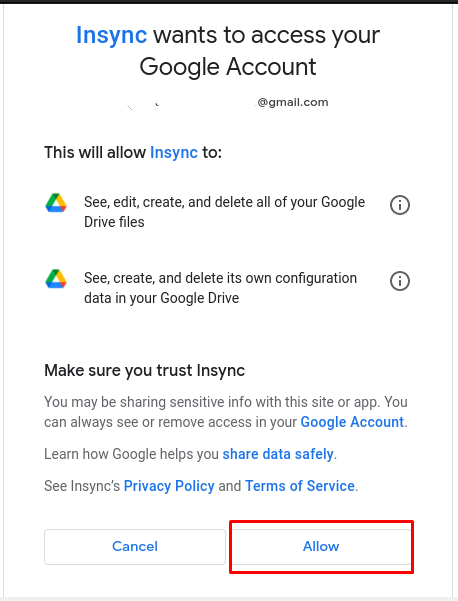The image features a notification set against a plain white background. At the top, there is a thin black horizontal line. Below this line, "NSYNC" is prominently displayed in blue text, followed by black text reading "wants to access your Google account." 

Further down, in black text, it says, "This will allow NSYNC," again with "NSYNC" in blue text, followed by a list of permissions: "see, edit, create, and delete all of your Google Drive files." Adjacent to this list is the Google Drive icon, depicted as a multicolored triangle.

Below this, another Google Drive icon appears, followed by the text, "see, create, and delete its own configuration data in your Google Drive."

In bold black text, you are advised to "Make sure you trust NSYNC." Below this, in light gray smaller text, a cautionary note reads: "You may be sharing sensitive info with this site or app. You can always see or remove access in your Google Account." The words "Google Account" are in blue and serve as a clickable link.

At the very bottom of the image are two action buttons: a gray "Cancel" button on the left and a blue "Allow" button on the right.